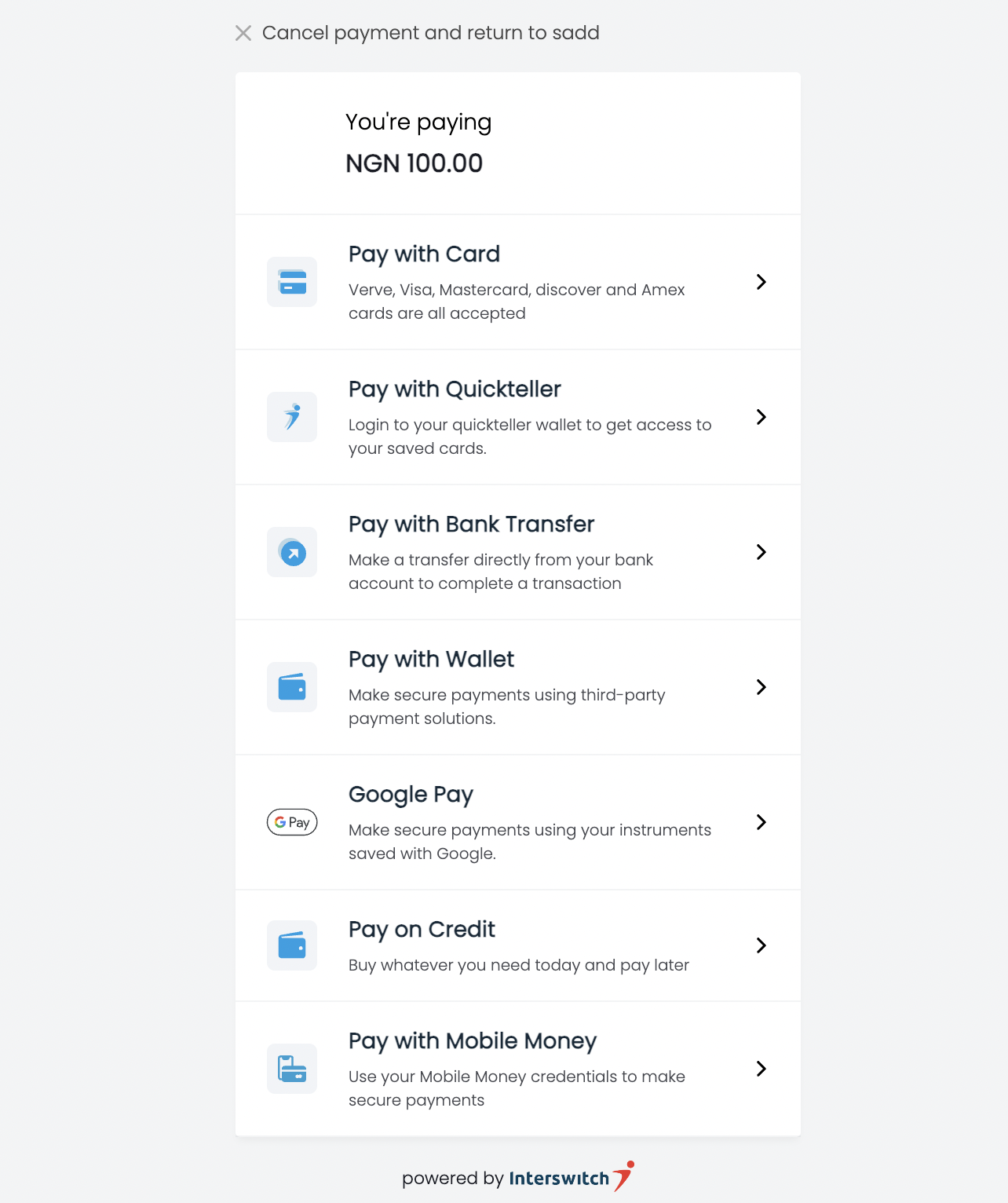The image displays a detailed screenshot of an online payment system, apparently from a website named SADD. At the top of the page, there is a small 'X' icon offering an option to cancel the payment and return to SADD. The user is currently set to pay a sum of NGN 100.

Several payment options are listed below:

1. **Pay with Card**: An icon of a blue credit card is shown. Accepted card types include Verve, Visa, MasterCard, Discover, and Amex.
2. **Pay with QuickTeller**: Users can log in to their QuickTeller wallet to access their saved cards.
3. **Pay with Bank Transfer**: This option allows users to complete the transaction by making a direct transfer from their bank account.
4. **Pay with Wallet**: Users can make secure payments using third-party payment solutions.
5. **Google Pay**: Secure payments can be completed using cards saved with Google.
6. **Pay on Credit**: This option allows users to make purchases and pay for them later.
7. **Pay with Mobile Money**: Users can utilize their mobile money credentials for secure transactions.

At the bottom of the page, there is a note indicating that the system is powered by InterSwitch, accompanied by a red logo resembling a person with arms outstretched behind them, as if flying.